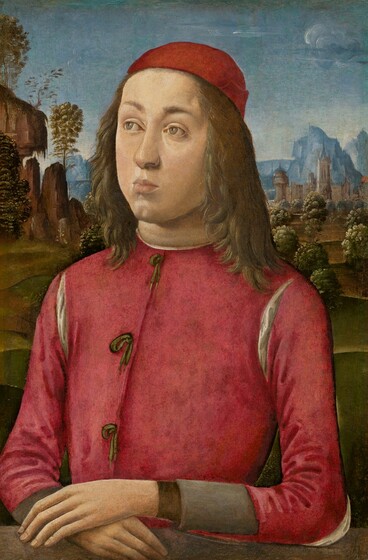The vertically aligned rectangular painting showcases a young man with a light complexion and long, feathery brown hair. He is wearing a detailed red uniform with white accents over the shoulders and brown cuffs adorned with gold trim. The uniform also has brown buttons running down the front. The man is also wearing a small, circular red cap atop his head. He is seated, with his arms crossed and resting on a brown surface, possibly a piece of wood. His expression is thoughtful, and his gaze is directed slightly off to the side as if deeply contemplating something significant.

In the background, a dark bluish-gray sky meets the outline of distant mountains and appears bright and clear with the day's lighting. Below the mountains, small round green plants add to the setting's natural beauty. To the left, there are brown rock structures contributing further to the serene landscape. This detailed scene paints a vivid picture of a contemplative individual in a serene natural environment.